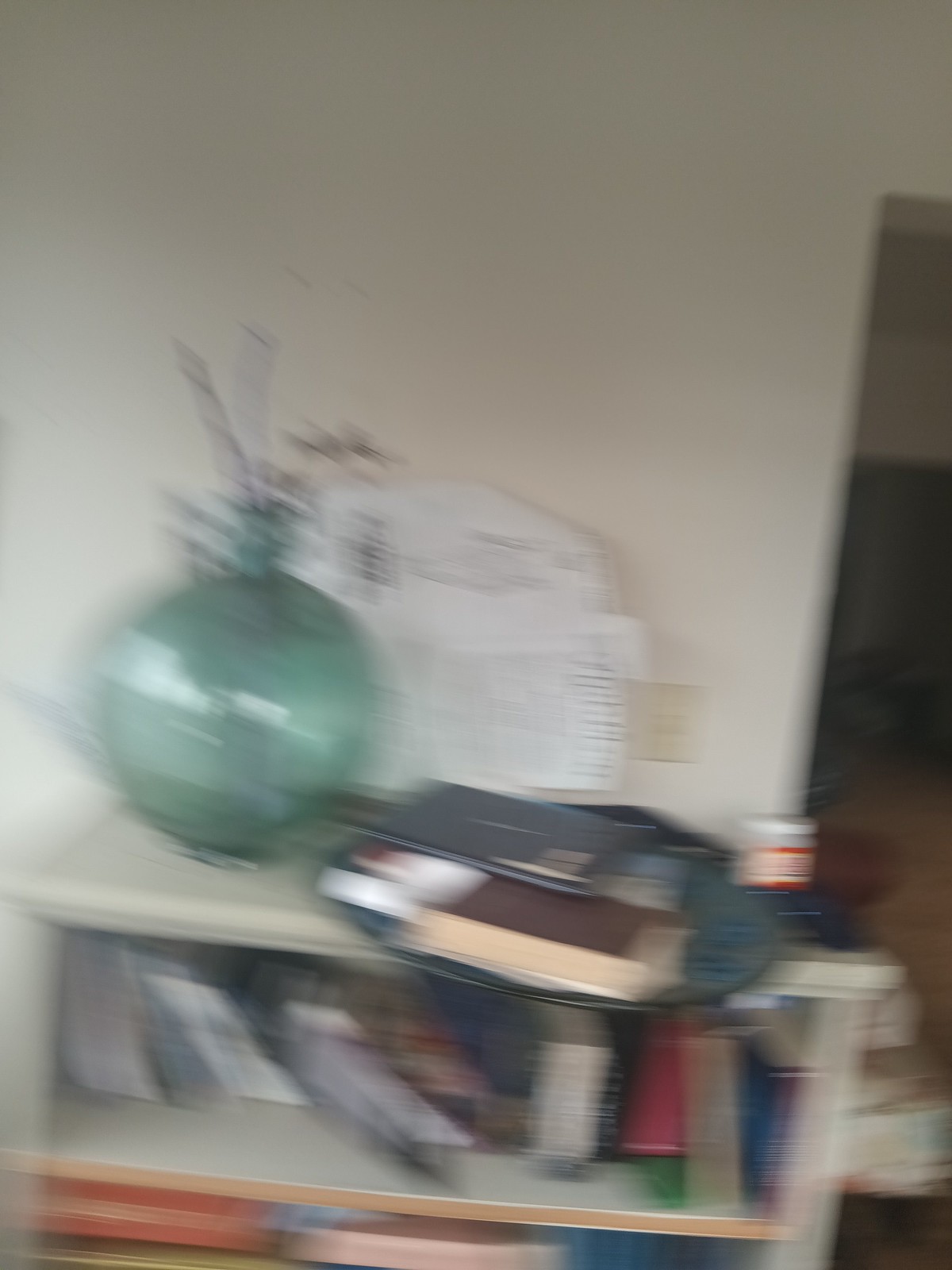This blurred image depicts a room with an off-white back wall, featuring a slightly yellowish portion at the bottom center, likely a light fixture. In the foreground, a short white bookcase with two shelves is apparent. Atop the bookcase to the left sits a large, round, green glass vase with a skinny neck, from which several branches or twigs protrude. Adjacent to the vase, there are indistinct objects, including a white item with a squarish base and a half-circle top, and brown and gray rectangular objects that may be books. On the lower shelves, there is an assortment of books or possibly software packages, though the exact details are unclear due to the blur. On the right side of the image, there is an opening leading to a walkway or hallway with a dark rectangle suggesting a doorway. Additionally, a sheet of white fabric or paper leans against the wall on the left side of the bookcase. The photograph's overall motion blur challenges clear identification of some objects.